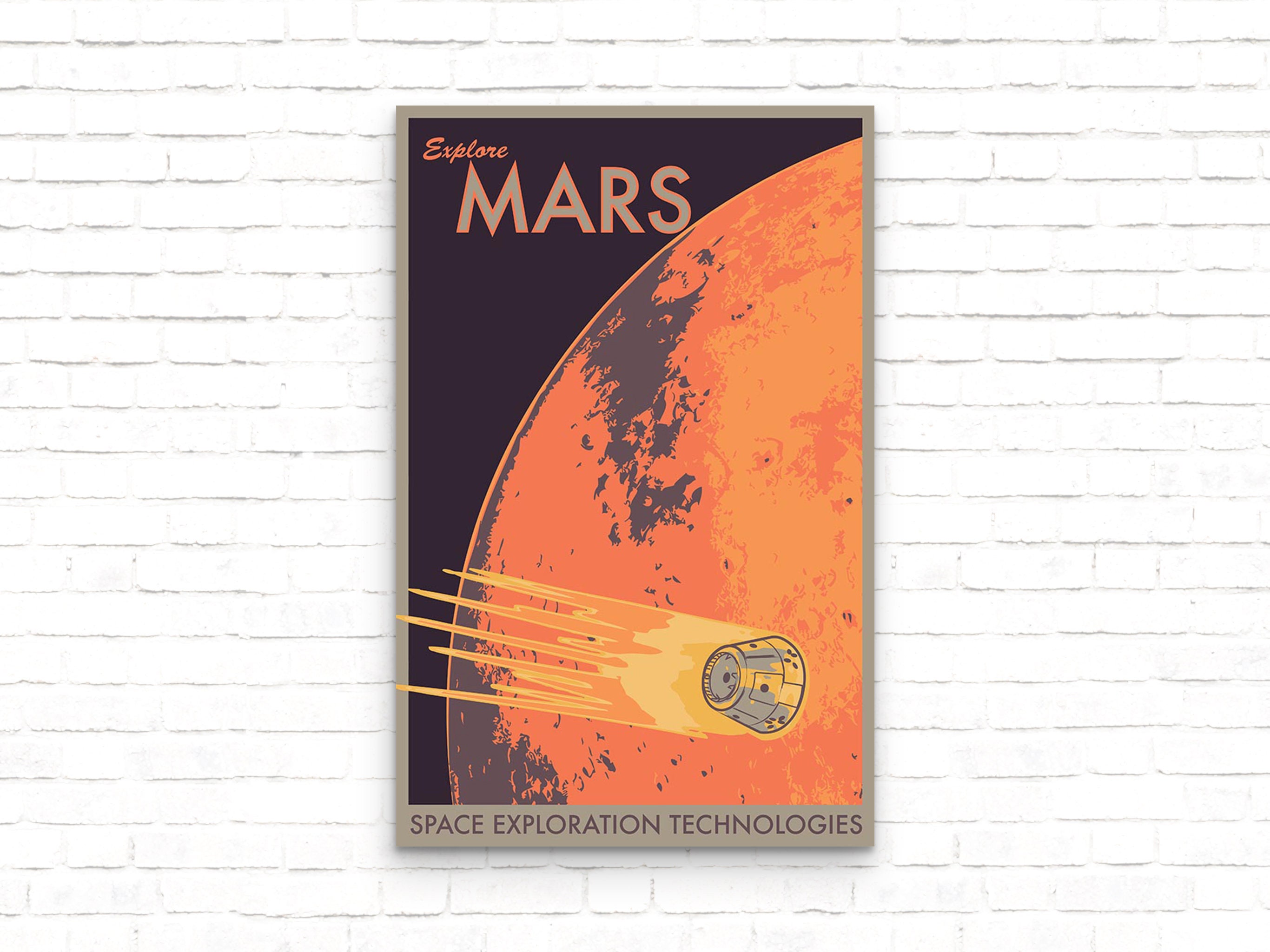The image depicts a digitally-rendered poster mounted on a generic white brick wall, likely designed as a conceptual piece for professional presentations or potential advertising campaigns. The poster features a deep brown, orange, medium brown, and dark bone color scheme. 

At the top left of the poster, the text "Explore Mars" is prominently displayed, with "Explore" written in a small, orange script font and "Mars" in large, gray block letters outlined in orange. The body of the poster showcases a close-up, partial view of Mars in vivid orange and gray hues, suggestive of the planet's rugged surface.

In the lower right corner of the poster is a triangular, gray spacecraft heading towards Mars, emitting a bright yellowish trail indicative of heat or propulsion. This dynamic effect is reinforced by movement lines extending into the poster's border. 

Completing the design, a beige border along the bottom of the poster displays the words "SPACE EXPLORATION TECHNOLOGIES" in bold, purplish letters. This evocative composition hints at ambitious space travel themes, potentially intended for movies, video games, or future marketing efforts.